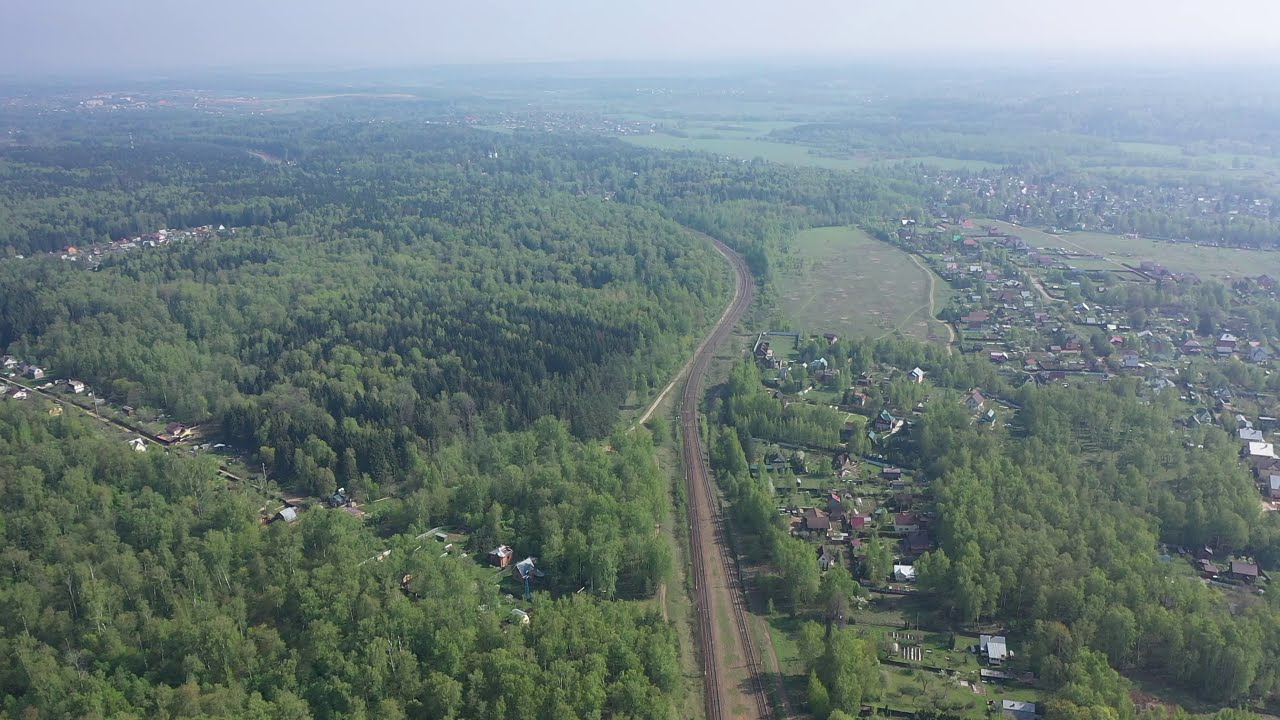This horizontal aerial photograph captures a rural and densely wooded area, predominantly filled with pine trees. The centerpiece of the image is a set of train tracks running through the small town, momentarily curving before vanishing into the thick forest which occupies the majority of the scene. The town is dispersed with houses and neighborhoods on either side of the tracks, with two-lane roads crossing over. In the foreground and middle of the image, several country homes with spacious plots and large lawns are scattered amidst the greenery. Small, interspersed clearings dot the landscape, with clusters of residential buildings peeking through the dense foliage. On the right side, more homes are visible, maintaining a rural, suburban feel. In the distant background, a serene lake snakes to the left, and beyond it, a mountain range capped with clouds frames the horizon. The overall impression is one of a tranquil, heavily forested countryside, intertwined with the modest spread of human habitation.